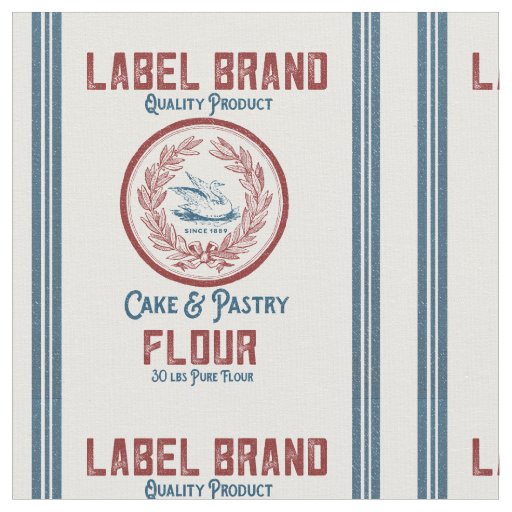The image depicts a square section of a packaging label with a light gray background. Prominently featured at the top is the brand name "Label Brand" in large red text, followed by "Quality Product" in blue text. Central to the design is a red circular emblem containing a blue swan with wings raised, encircled by a red crest and the text "Since 1859" in small lettering. Below the emblem, the words "Cake and Pastry" appear in blue text and are followed by "Flour" in large red text. Further down, "30 pounds pure flour" is written in small blue text. The entire design is framed by blue vertical lines along both sides, repeating to create a symmetrical border. The text and lines appear slightly faded, creating a vintage look.